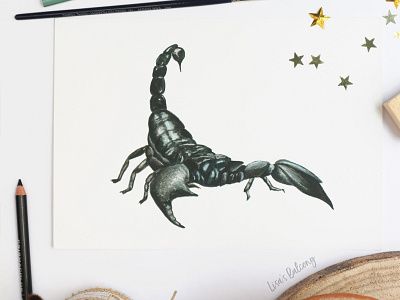This photograph captures a detailed drawing of a scorpion on a piece of white paper lying on a white table. The scorpion, meticulously rendered in charcoal or black colored pencil, is oriented with its tail raised and poised as if ready to strike, while its claws are extended towards the viewer. To the top right of the drawing, gold star confetti is scattered, adding a touch of color to the monochromatic illustration. A sharpened black colored pencil is placed to the left of the paper, partially visible. In the foreground, the edge of a circular wooden object, possibly a coaster, peeks into the frame. The artist's signature, "Lisa Belong" or a similar variation, is inscribed at the bottom of the drawing, marking the piece as a creation by Lisa.